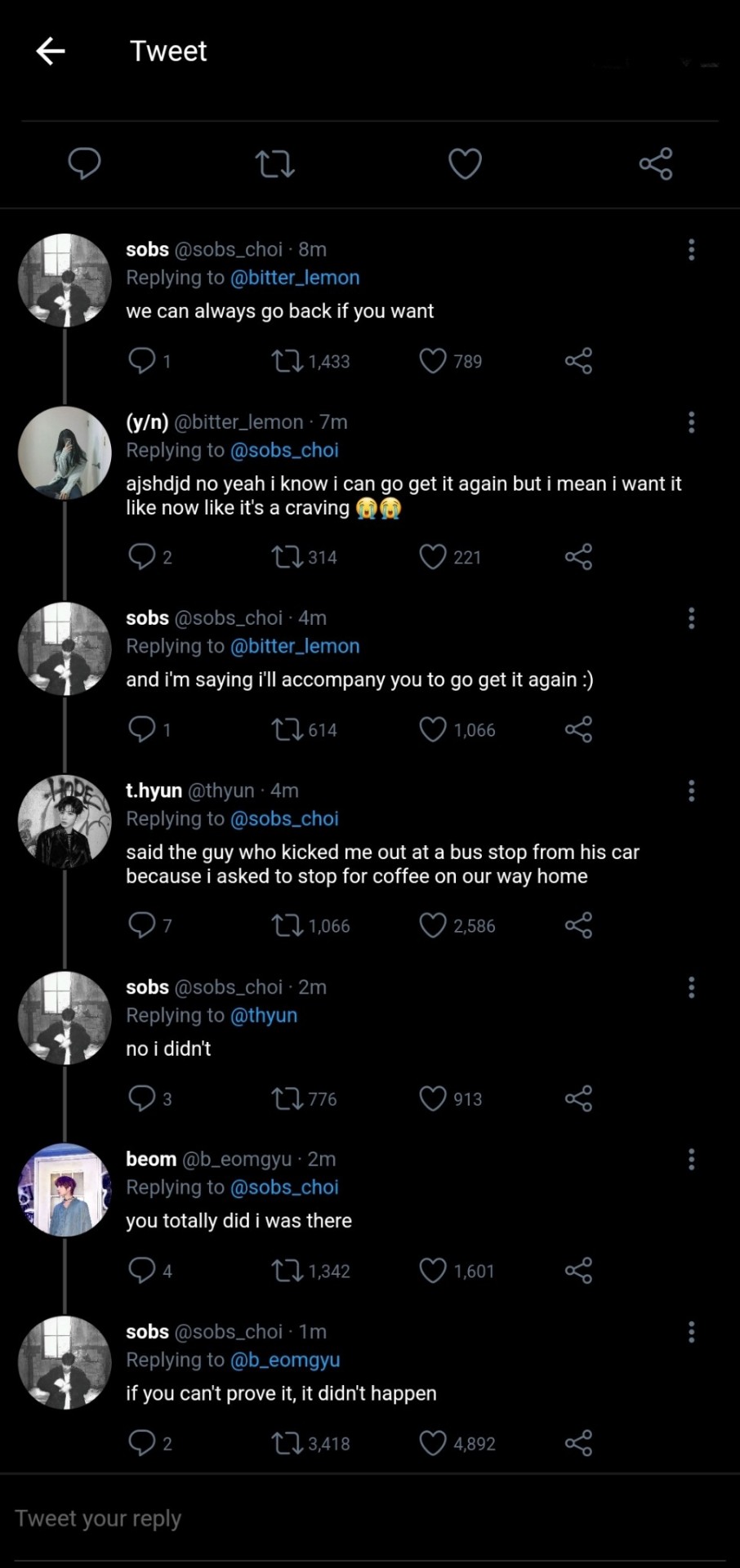The image displays an animated conversation on Twitter among several users, prominently led by a user named Sobs. The dialogue unfolds as follows:

- **Sobs** initiates the thread with a tweet: "We can always go back if you want."
- **Bitter Lemon** promptly responds with their thoughts, followed by a reply from **Sobs**.
- **Thian** joins the conversation with a comment, to which **Sobs** again responds.
- Subsequently, **Bion** contributes to the thread, and **Sobs** replies once more.

The interaction appears to be predominantly driven by Sobs, who is the most active participant. 

The avatars of the users display Asian faces, suggesting that the participants are from Asia. Additionally, some usernames and cultural references, such as **Bitter Lemon**, commonly found in Japanese context (including songs), hint at a possible Japanese background of the users. 

This lively exchange reflects the typical flow of communication on social media, likely Twitter, showcasing a blend of cultural nuances and digital interaction.